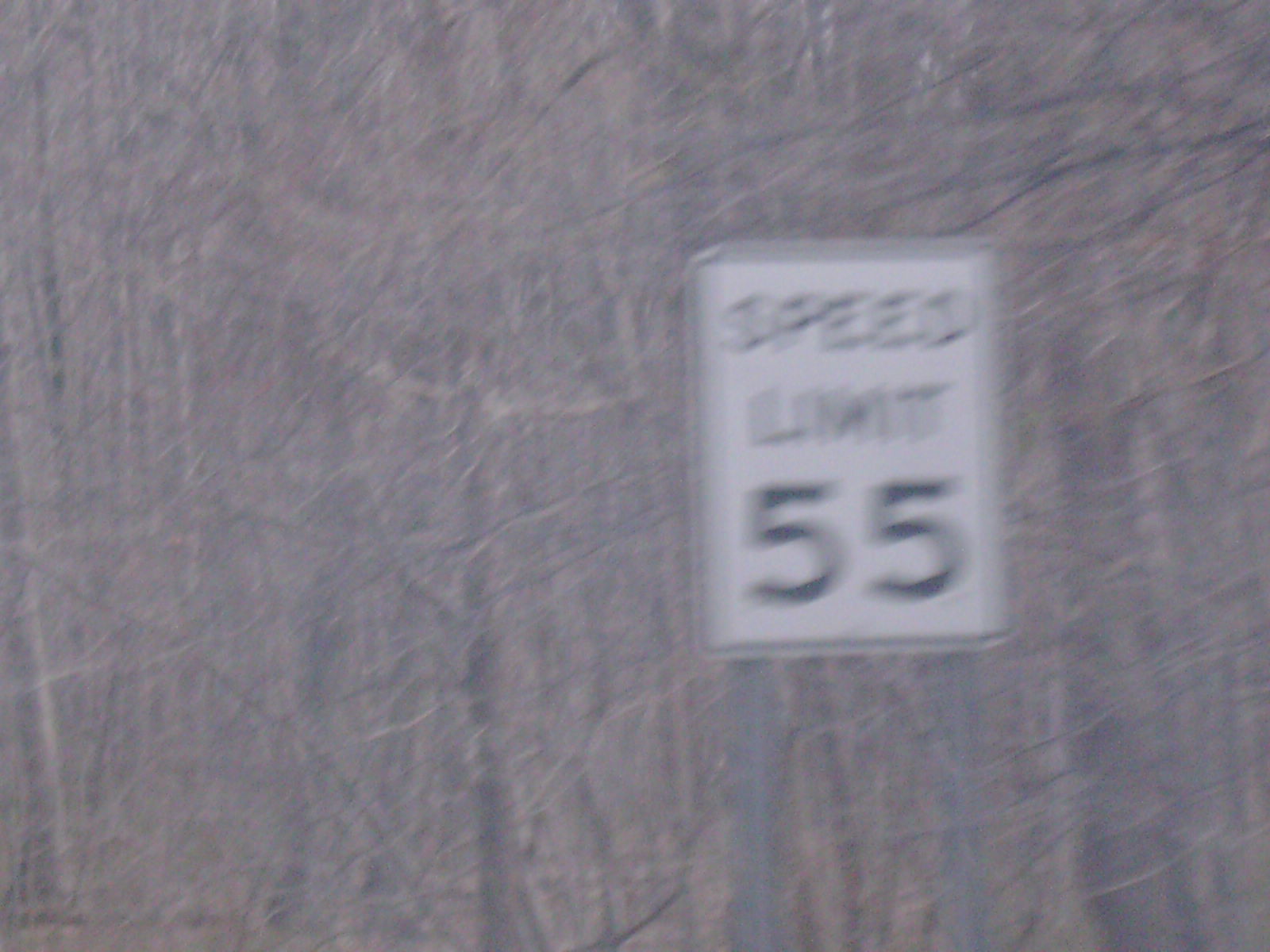A white rectangular speed limit sign with black lettering indicating a speed limit of 55 mph is prominently featured in the foreground, mounted on an aluminum stake. The words "Speed Limit" are slightly blurred, but the number "55" is clear and easily readable. Behind the sign is a densely wooded area with a mix of brown trunks and branches, which suggests a forest environment. The entire image is somewhat blurry, indicating that it might have been taken from a moving vehicle. There is a hint of morning light, visible as a grayish hue in the background, adding to the early-day ambiance. Although there are no visible roads or other structures in the frame, the overall scene suggests a rural or semi-rural setting. Scattered leaves and small branches are also visible at the base of the sign, further emphasizing the natural surroundings.